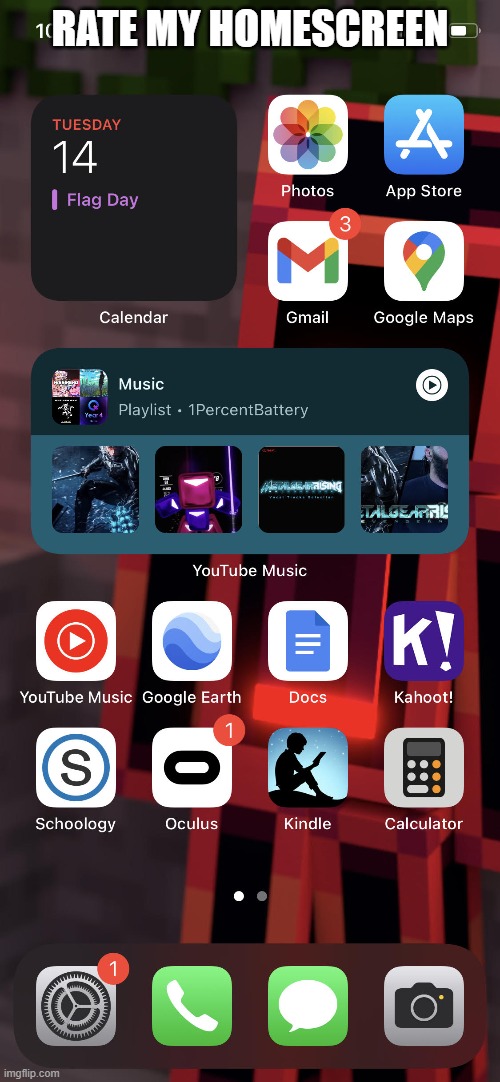This image is a detailed screenshot taken from a mobile device, showcasing a personalized home screen. At the very top, overlaid text reads "Rate my home screen," suggesting a prompt for feedback. The bottom of the screen features a visible watermark from imgflip.com, indicating the source of the screenshot.

The home screen is organized with a navigational bar at the bottom, including icons for settings, making phone calls, sending messages, and opening the camera. Prominently, there is a date widget for quick reference, as well as a YouTube Music widget that allows the user to play music directly from the home screen.

The user’s app icons are neatly arranged and include shortcuts to Photos, App Store, Gmail, Google Maps, YouTube Music, Google Earth, Docs, Kahoot, Schoology, Oculus, Kindle, and Calculator. The background image is a striking red and black abstract design, resembling a robot, adding a unique visual appeal to the home screen.